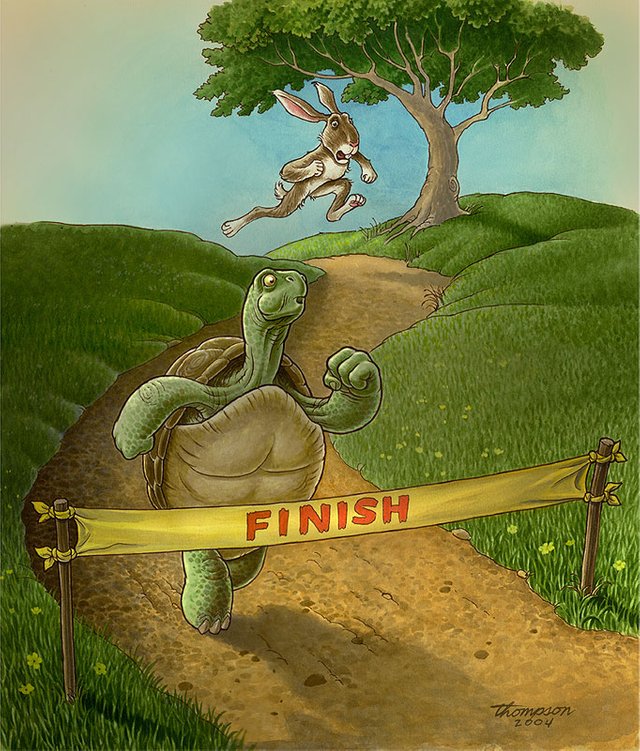In this semi-realistic cartoon illustration depicting the climactic moment of the children's story "The Tortoise and the Hare," we see a vividly detailed race scene. The tortoise, green with a brown shell, is running on two feet and breathing heavily as it approaches the finish line, only one or two steps away. The finish line is clearly marked by a ribbon tied across two sticks placed on either side of the brown pathway. The word "FINISH" is prominently displayed in red ink on the banner. Right behind the tortoise, we see the distressed hare, brown with white underparts and long ears trailing behind. The hare is also running on two feet, trying to catch up but visibly alarmed by the likelihood of losing. The scene is set against a background featuring a single tree, green grass bordering the pathway, and a blue sky, indicating daytime. In the bottom right corner of the image, the artist's signature, "Thompson 2004," is scribbled.